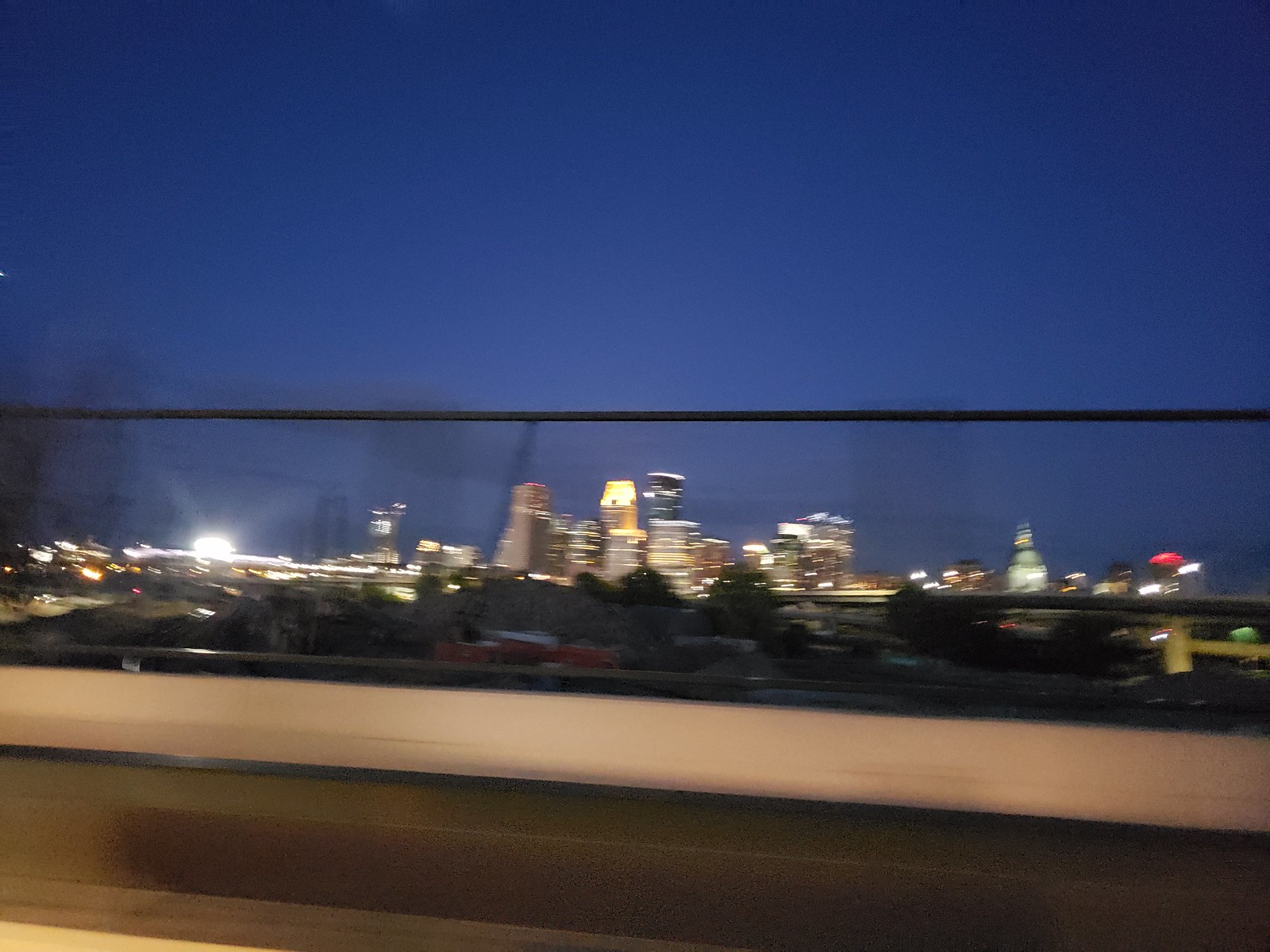Captured during the night, this photograph presents a blurry vista of a city skyline against a deep blue sky. Dominating the center of the image is a horizontal black line, under which the luminous cityscape emerges. Buildings of varying heights, adorned with lights, populate the scene. Prominently, a tall white-lit building stands to the right, flanked by shorter edifices. To the left, additional buildings are visible, accompanied by a striking bright white light. In the foreground, the tops of trees obscure part of the view, with a broad white horizontal rectangle just below them. The lower portion of the image dissolves into a blurry mix of gray and brown tones, implying the photo was taken from the window of a slowly moving car.